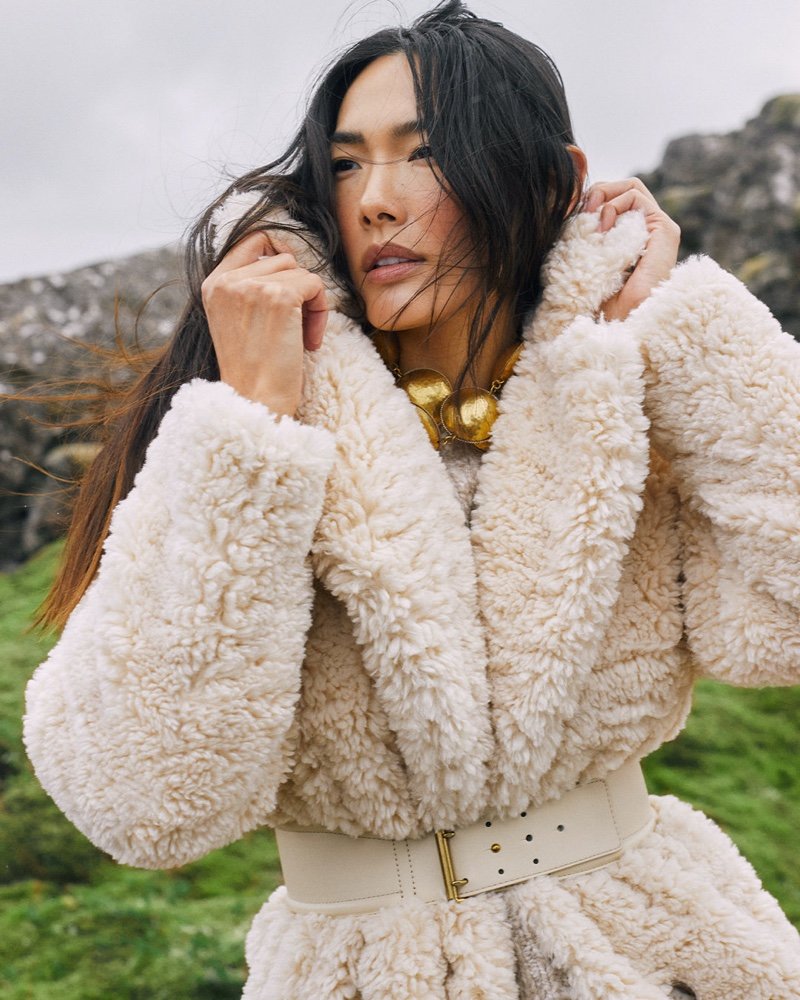This is a realistic, vertical color photograph set outdoors featuring a striking scene. In the background, a light gray sky looms over a diagonal spread of gray rocks extending from the top right to the center left of the image. Dark trees and foliage are subtly present, hinting at a serene, natural environment. The middle ground reveals a lush patch of green grass, slightly out of focus, enhancing the depth of field and bringing the subject into sharp clarity.

The central focus of the photograph is a woman, possibly in her 20s, with a blend of Native American or East Asian-Japanese features. She possesses light skin, an angular face, and long black hair that transitions into a burnt orange hue at the tips. The woman's attire is notably stylish and chic, suggesting a fashion model presence. 

She wears a voluminous, fuzzy white coat with pronounced lapels and a substantial collar, clinched at her waist with a beige leather belt featuring a double-pronged gold buckle. Her hands are actively engaged with her coat; her right hand clutches the collar tightly, while her left hand is raised, fingers curled as if adjusting to the chilly or windy weather. She is adorned with a striking gold necklace composed of large, spherical gold baubles, adding a touch of glamour to her ensemble.

The woman stands confidently amidst the green hillside, facing forward but gazing towards the left side of the frame. Her demeanor, combined with the dynamic setting, creates a compelling and visually captivating scene devoid of any text annotations.